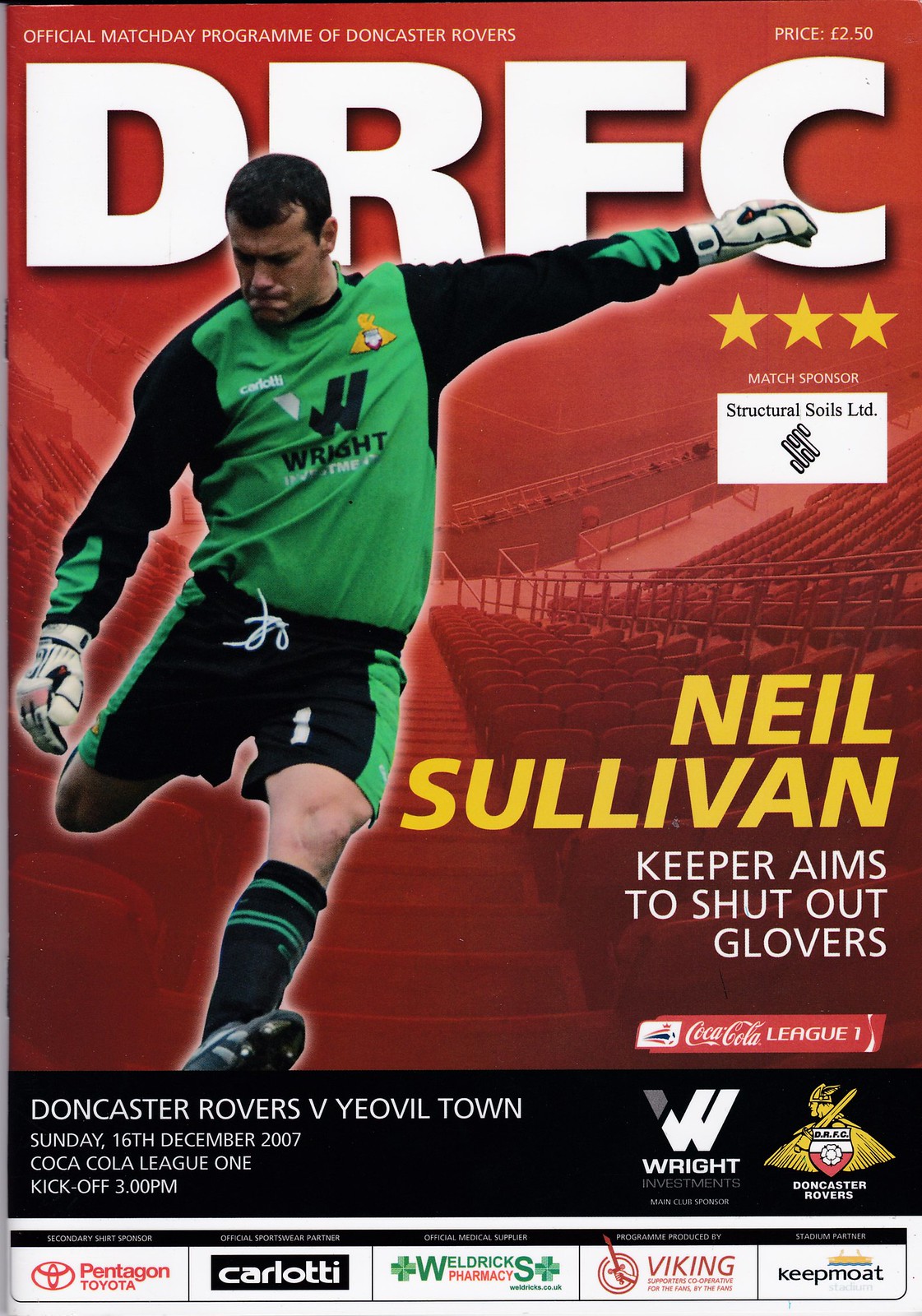The image is the cover of an official match day program for Doncaster Rovers, priced at £2.50. The magazine, titled "DRFC," prominently features a dynamic photograph of Neil Sullivan, the keeper, in a green uniform with black sleeves, poised to kick a soccer ball. The background displays a stadium with empty red seats on the right. Text on the cover reads, "Official Match Day Program of Doncaster Rovers," and highlights Neil Sullivan with the caption, "Keeper aims to shut out Glovers."

Below, additional text states, "Match Sponsors: Structural Soils Limited" and features the Coca-Cola League One logo. In a black bar at the bottom, the text details the match event: "Doncaster Rovers versus Yeovil Town, Sunday, 16 December 2007, Coca-Cola League One, kickoff 3pm." The right side of the bar includes the Wright Investments logo and the Doncaster Rovers emblem, depicting a Viking with a shield and sword.

Supporting sponsors listed at the bottom are Pentagon, Toyota, Carlotti, Weldrick Pharmacy, Viking, and Keepmoat.